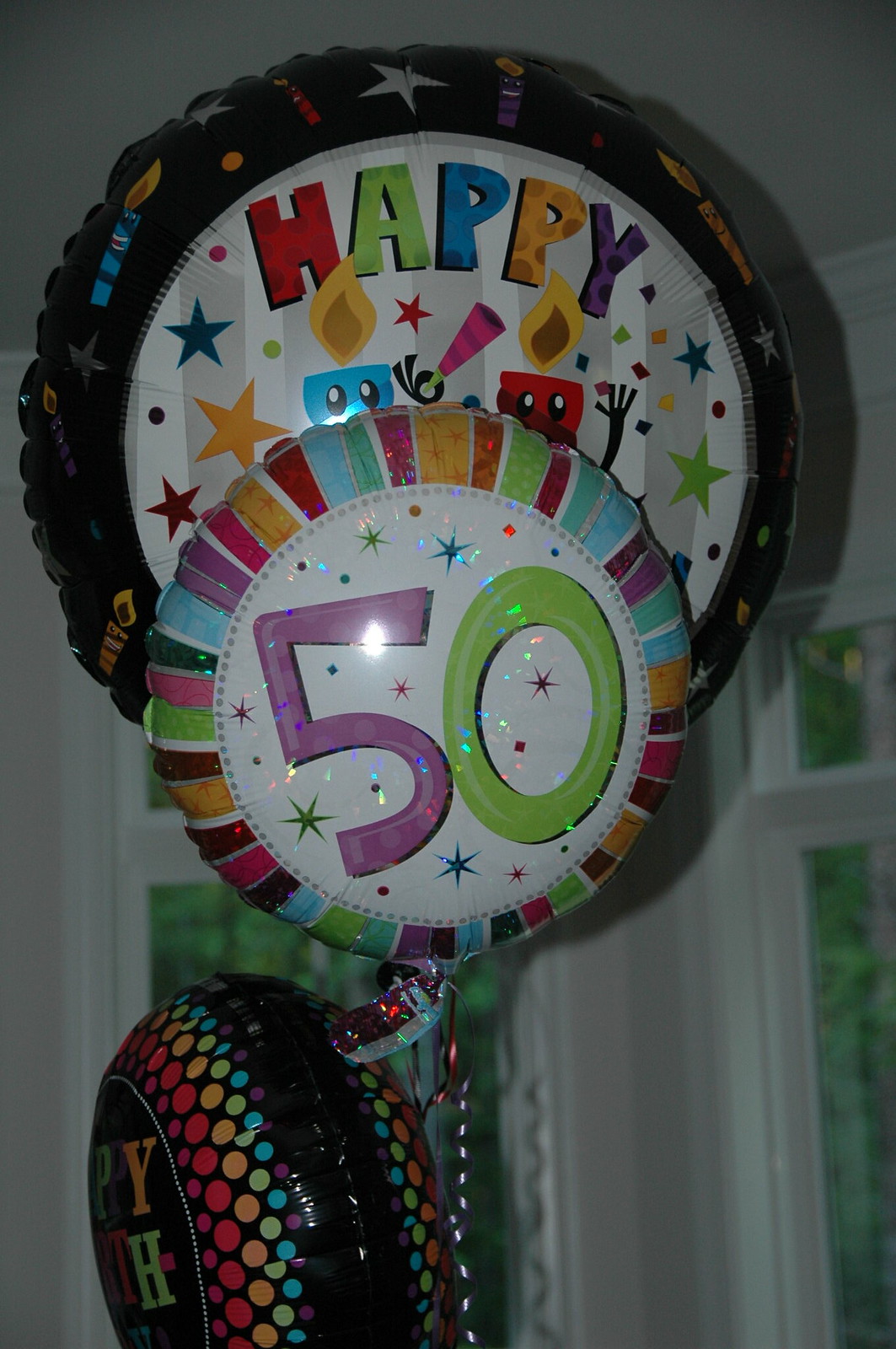This photograph captures a trio of colorful celebratory balloons floating in a living room against a backdrop of white walls and windows, indicating a cozy indoor space. The largest balloon proudly displays the festive message "Happy Birthday" in various vibrant colors, adorned with celebratory confetti, stars, and playful elements like candle figures with eyes and arms. Foregrounded and partially covering the birthday balloon is a striking number "50" balloon, with the numeral "5" in purple and "0" in green, suggesting a milestone 50th birthday celebration. A third balloon, smaller and darker, peeks from the side, characterized by its black surface dotted with multicolored spots. Despite the gathering dusk visible through the windows, the balloons buoyantly float upwards, tethered to a base, yet reaching for the ceiling, encapsulating the joyous spirit of the occasion.